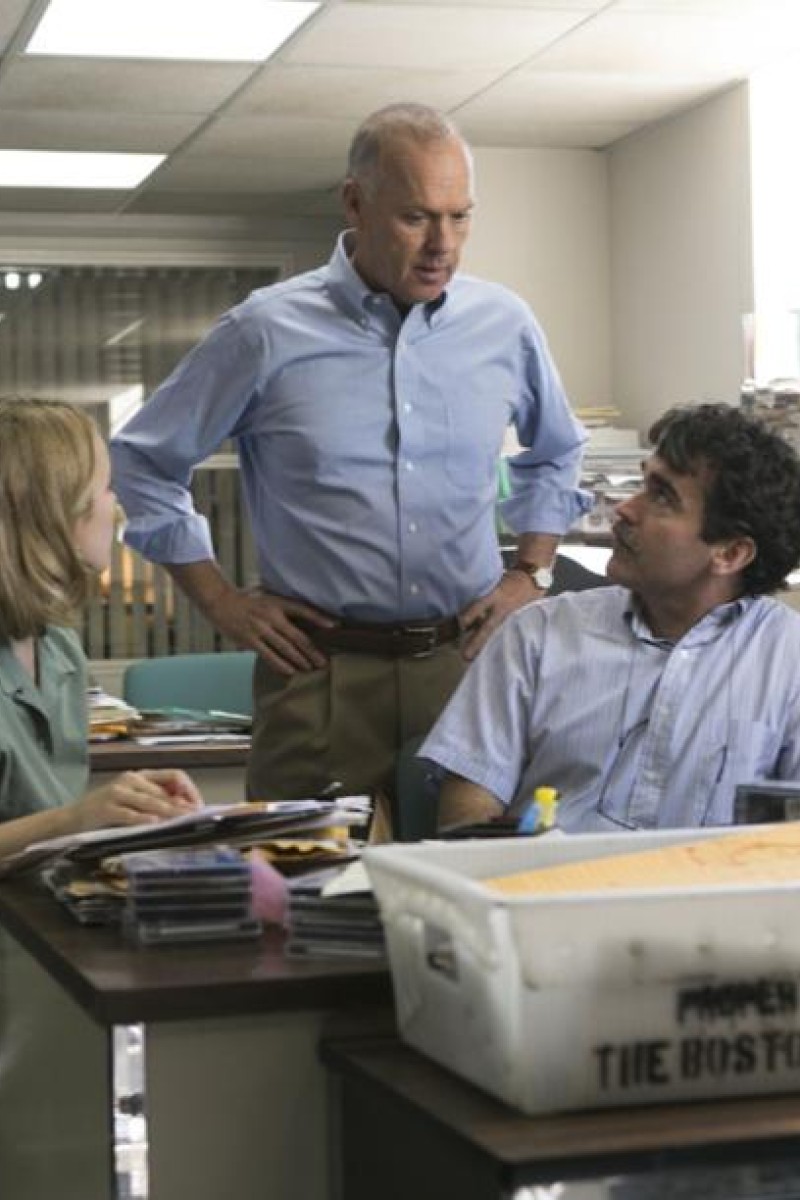In this digital or film photograph set in an office, three individuals are captured in a moment that suggests a workplace dynamic. At the center stands an older, mostly bald man with a greyish hue to his remaining hair. He exudes an air of authority, with his hands firmly placed on his hips. He is dressed in a long-sleeve blue button-up shirt, tan khaki pants, and a brown belt, complete with a watch on his left wrist. He is likely a boss or supervisor.

To the right of the image, sitting at a brown wooden desk cluttered with CDs and packages, is a white man with longer dark curly hair and a mustache. He wears a blue short-sleeve button-up shirt and has glasses hanging from his neck, indicating he might be an employee or subordinate to the standing man.

On the left side of the image is a blonde woman with short hair, possibly wearing green scrubs, suggesting she might have a different role in the workplace. She gazes up at the man standing, which reinforces the impression of his authoritative position. The office environment is characterized by white walls and a white ceiling lit by overhead lights. This setting and the individuals' attire and postures collectively create a clear depiction of a boss engaging with his team in a workplace scenario.